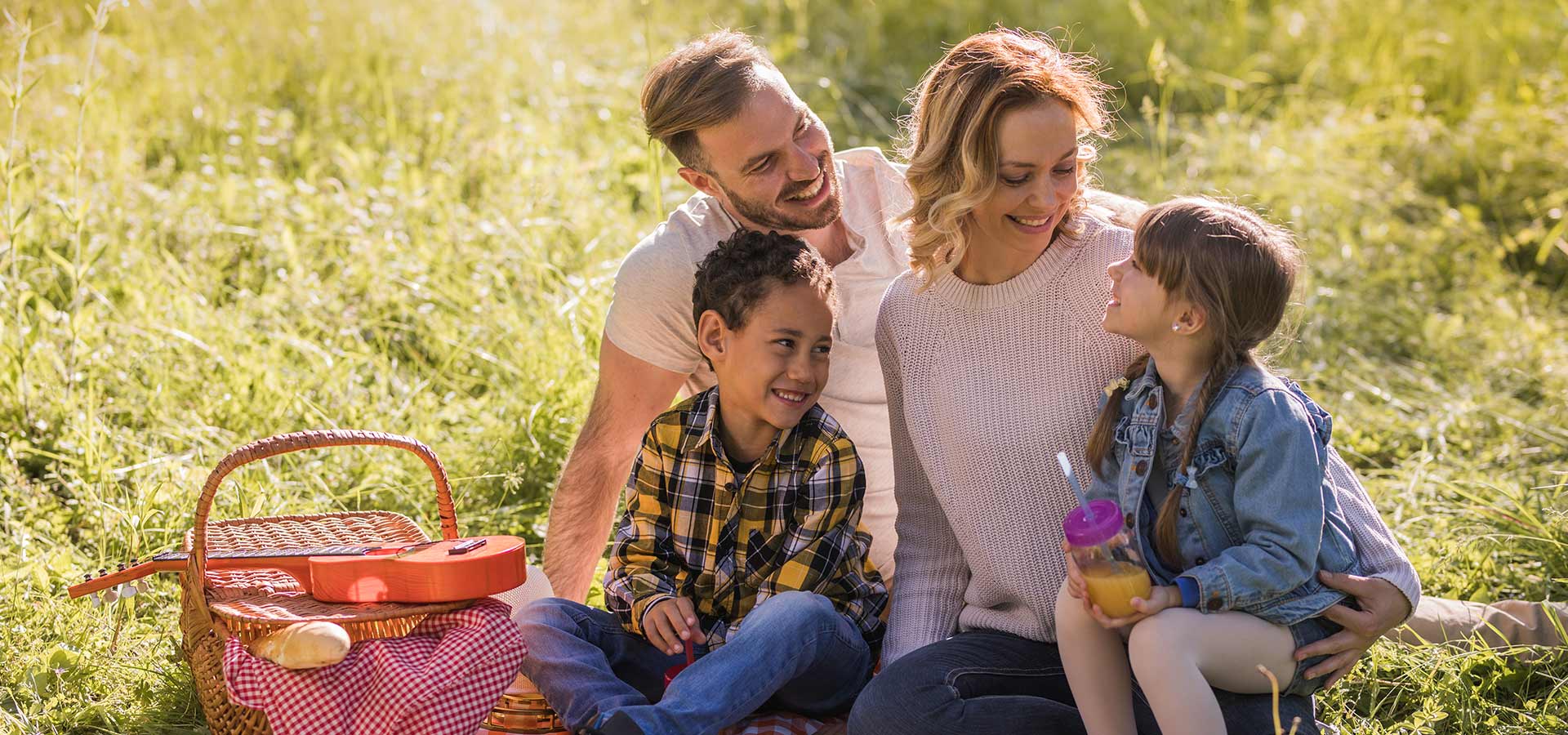In this serene outdoor photograph, a joyful family of four enjoys a sunny picnic in a meadow with lush, unmowed grass. The parents, a smiling couple in their 30s, are seated with their two children—a boy and a girl. The father, clad in a white shirt with light brown hair and a beard, holds the boy who wears a plaid checkered shirt and blue jeans. The boy's fingers gently hold the straw of a cup. The mother, dressed in a beige sweater and jeans, has curled blonde hair and warmly cradles the daughter on her lap. This young girl, with brown hair styled in pigtails and bangs, smiles at her father while holding a cup of orange juice with a blue straw. She wears a denim jacket and tights.

To their side, a wicker picnic basket adds a charming touch to the scene, with a loaf of French bread peeking out and a small mandolin or toy guitar placed on top. A classic red and white checkered picnic blanket is also tucked into the basket. The sunlight bathes the family, highlighting their happy expressions as they share this picturesque and heartwarming moment.